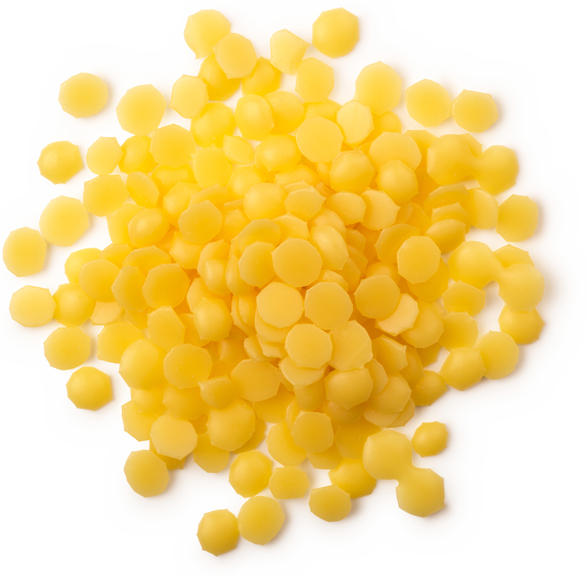The image features a multitude of small, yellow, roundish pieces, densely concentrated in the center and becoming sparser towards the edges, forming an imperfect circular shape. The background is entirely white, emphasizing the vibrant yellow of the objects, which could be mistaken for either candy, plastic bits, pills, or even frozen corn. The specific nature of these items is ambiguous, adding an intriguing element to the photo. The lack of text and the stark, nondescript background make it challenging to pinpoint the setting, leaving open the possibility that this scene could be located in various environments, such as a doctor's office, a home, or a business. The arrangement of items suggests they were simply scattered or dumped onto the surface.